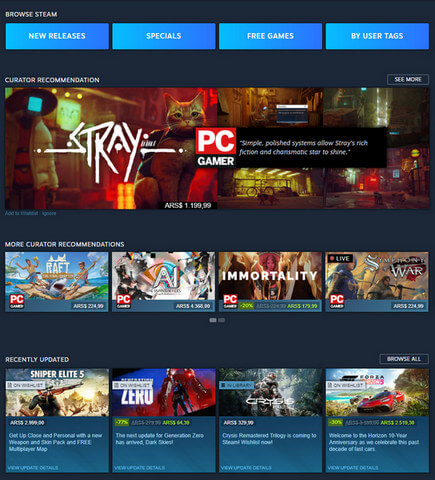The image features a user interface screen from a gaming platform with a dark gray background at the top left. Prominently displayed in white capital letters are the words "BROWSE STEAM." Below this heading, there are four light blue rectangular boxes arranged horizontally, labeled from left to right as "New Releases," "Specials," "Free Games," and "Browse User Tags." Beneath these boxes, another section titled "Curator Recommendations" is presented, accompanied by a "See More" button.

In the "Curator Recommendations" section, a small, intricate image appears, depicting a steampunk-inspired background with the picture of a cat. Although the details of the image are somewhat unclear, the text next to it reads: "Stray PC game: Our simple, polished system allows Stray’s rich fiction and charismatic characters to shine."

Further down, a section labeled "More Curator Recommendations" displays a list of games, including "The Rav," "AI," and "Immortality." Below this list, another section titled "Recently Updated" highlights the game "Sniper Elite 5." On the far right side of the screen, there is an image from a racing game showing a red car navigating a turn at high speed.